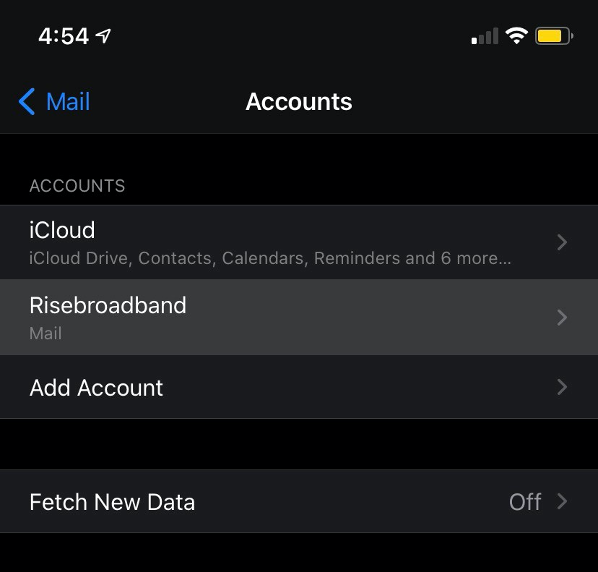This image appears to be a screenshot taken from the settings section of a smartphone. At the top right of the image, there's a battery icon colored yellow, indicating about 80% charge. Left of the battery icon is a Wi-Fi symbol with four bars, and to its left is a phone signal icon showing one full bar. At the top left, the time is displayed as 4:54, accompanied by a location icon shaped like an arrow pointing to the top right.

In the top middle of the screen, the word "Accounts" is prominently displayed. To its far left, the word "Mail" accompanied by a left-pointing arrow is highlighted in blue.

A list of items is visible starting from the far middle left of the screen. The first item is "Accounts," followed by "iCloud," "Rise Broadband," and "Add Account." Under the "iCloud" section, there is a sub-list featuring "iCloud Drive," "Contacts," "Calendars," "Reminders," and other categories totaling six more, each with a right-facing arrow next to them.

At the bottom left, the phrase "Fetch New Data" is visible, with the option status labeled as "Off" and accompanied by a right-facing arrow.